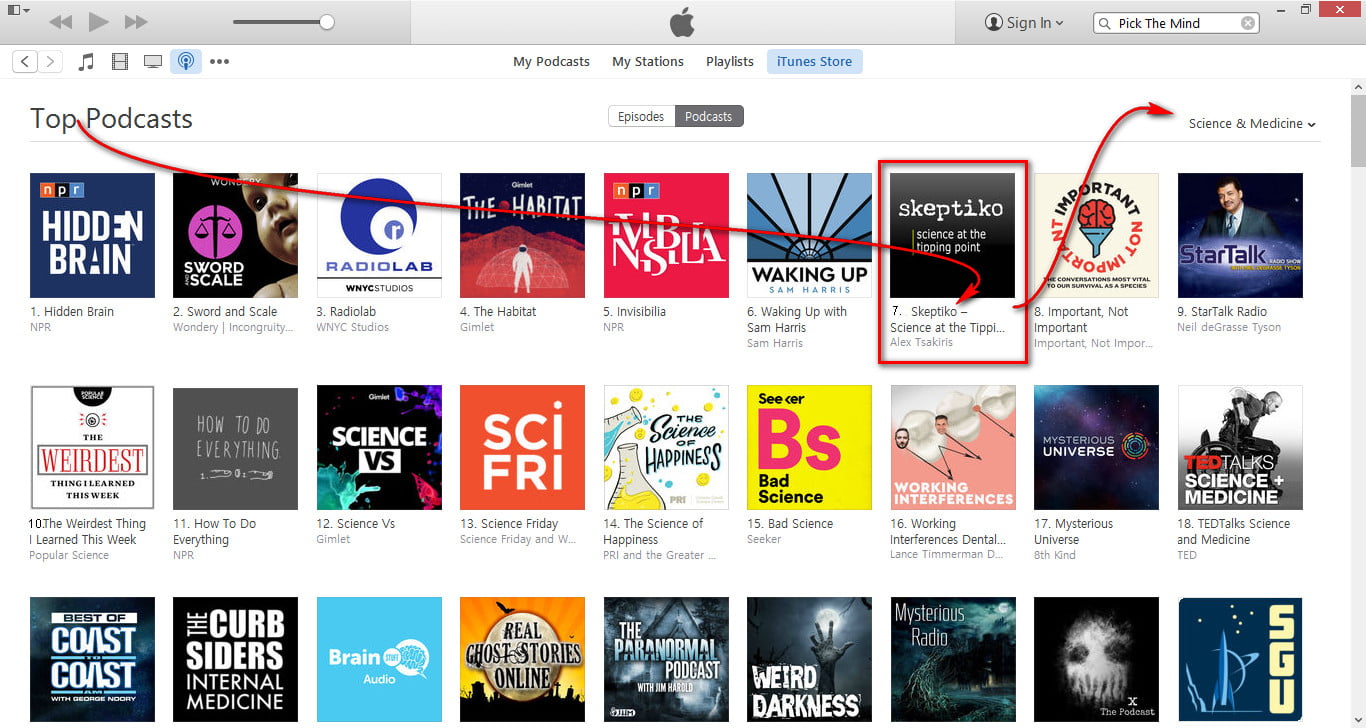The screenshot displays the iTunes interface, specifically within the iTunes Store tab, under the Podcasts section. The user has navigated to the Science and Medicine genre, showcasing a variety of science-related podcasts. Visible tabs at the top include "My Podcasts," "My Stations," "Playlists," and "iTunes Store." The highlighted podcasts include notable titles such as "NPR Hidden Brain," "V-Lab," "Invisibilia," "StarTalk with Neil deGrasse Tyson," "Skeptico," "Bad Science," "Science Friday," and "Science Versus," among others. The general window has a white background, with a search bar located in the top-right corner. Arrows have been added to indicate the podcast "Skeptico" and the genre selector.